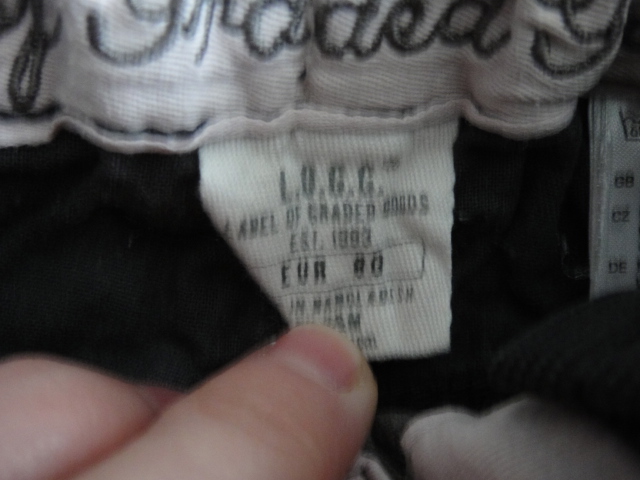In this image, a Caucasian hand with short, pink nails is prominently displayed, holding a white tag affixed to a garment made of black fabric. The hand is pointing towards the tag, which reads "L-O-G-G," followed by "Label of Graded Goods" and "Established 1993." The text also includes "EUR 80" and "Made in Bangladesh," though parts of it appear blurred. Above this smaller tag is a larger, white rectangular tag with unreadable lettering or a logo, partially obscured and embroidered. The close-up nature of the photograph highlights the details of the tags and hand but makes the type of clothing difficult to identify.